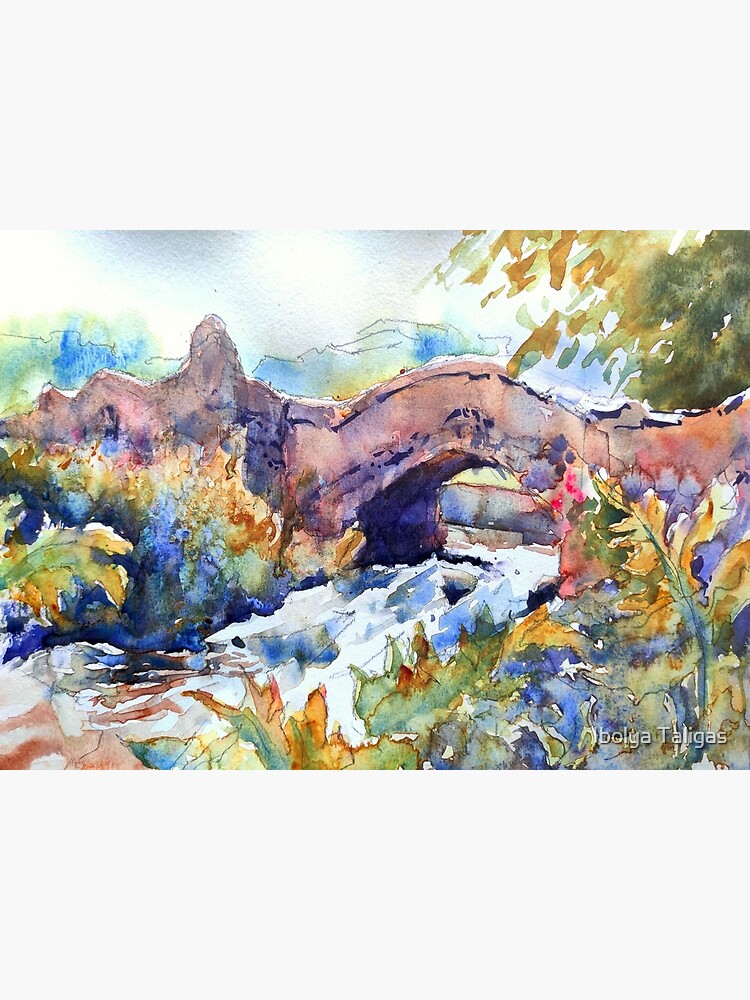This detailed watercolor painting, titled "BOLYA TALIGAS" as signed at the bottom, showcases a serene outdoor landscape with broad, impressionistic strokes. Central to the image is an adobe-colored stone bridge arched gracefully over a blue and white, rough-flowing creek, or small river, which winds out of the frame to the right. The bridge, possibly leading to a distant village, incorporates both a walkway and a stone rail. On either side of the water, lush green foliage, grass, and an array of flowers provide a vibrant foreground.

To the right of the bridge, a tree with darker green hues stands prominently, its branches and leaves overhanging the scene. Similarly, the left side boasts more trees and a colorful array of plants with hints of gold and yellow, adding to the textured landscape. Further back, the outline of a mountain range is subtly suggested in shades of green, blue, and gray, adding depth to the horizon. Above, the sky is painted in gradient tones with gray at the top descending into white, fluffy clouds. The entire scene, rich with natural detail, from flowing water to textured flora, effectively captures the essence of a tranquil and picturesque countryside.